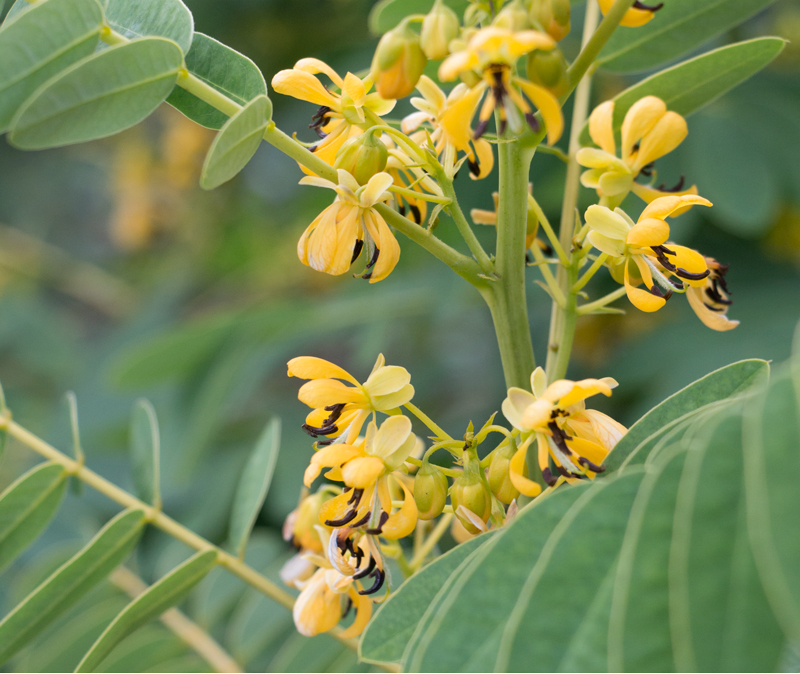This is a detailed close-up daytime photograph of a cluster of delicate yellow flowers. The central focus is slightly to the right of the image, with a prominent green stalk adorned by 10 to 12 elongated yellow buds, most of which have bloomed. Each vibrant flower has long, drooping petals and stamens ending in tiny black specks. Surrounding the flowers are light green, oval-shaped leaves with clearly visible veins. In the foreground to the right, there is a broad green leaf that's slightly out of focus. To the lower left, a diagonal stem features six narrow green petals. The background features a blurred blend of bluish and green tones, drawing attention to the intricate details of the yellow blossoms and the green stems.